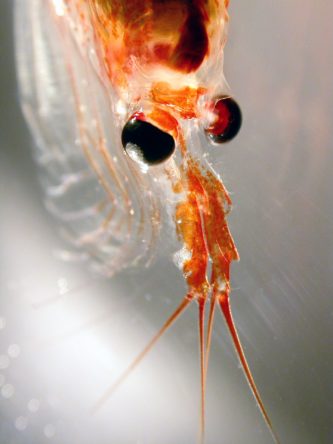This detailed image captures a vibrant orange shrimp set against a minimalist gray background. The shrimp's body displays shades of orange and dark orange, with a translucent quality to its form. Dominating the image are its prominent black bulging eyes, each with unique characteristics—one eye is primarily black with a white center, while the other has a mix of red and black. Emerging from the shrimp's face are four long, whisker-like appendages that add to its distinctive appearance. The shrimp is positioned descending from the top middle of the image, with its tail possibly curling underneath its body. The overall scene presents the shrimp with clarity, highlighting the fine details and textures of its anatomy.